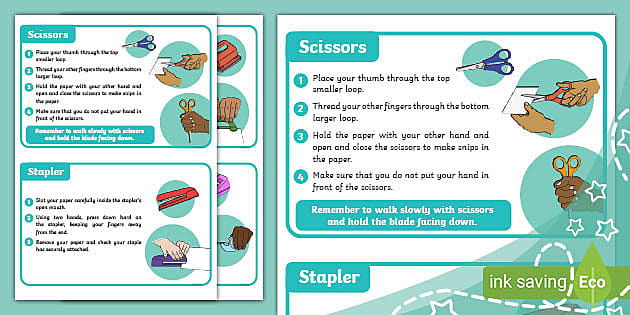This educational poster, predominantly in blue and brown hues with a substantial white background, is centered on the proper use of scissors. The layout is neatly divided in the middle, featuring a panel on the upper left side.

In the upper left corner of the blue panel, bold white letters spell out "Scissors." Adjacent to this text is a circle containing a detailed illustration of a pair of scissors. Following this, another drawing depicts two hands using the scissors to cut a piece of paper, emphasizing the correct hand positioning and technique. Below this, an image shows a hand holding the scissors upright by its blades.

Beneath the blue section, a set of instructions in white letters offers a step-by-step guide on using scissors safely: 

1. Place your thumb through the top smaller loop.
2. Thread your fingers through the bottom larger loop.
3. Hold the paper with your other hand.
4. Open and close the scissors to make cuts.
5. Ensure that you do not put your hand in front of the scissors.

Further down, another reminder in white text against the light blue background advises: "Remember, we walk slowly with scissors and hold the blade facing down."

To the left, similar symbols and instructions are presented, including the word "Scissors" in another language, showcased in smaller print.

In the bottom right corner, the phrase "Ink Saving ECO" is printed in white letters on a green background, indicating the poster's eco-friendly ink usage. Just to the left, the term "Stapler" appears in white against a light blue background, hinting at a related topic for safe and efficient use of common office tools.